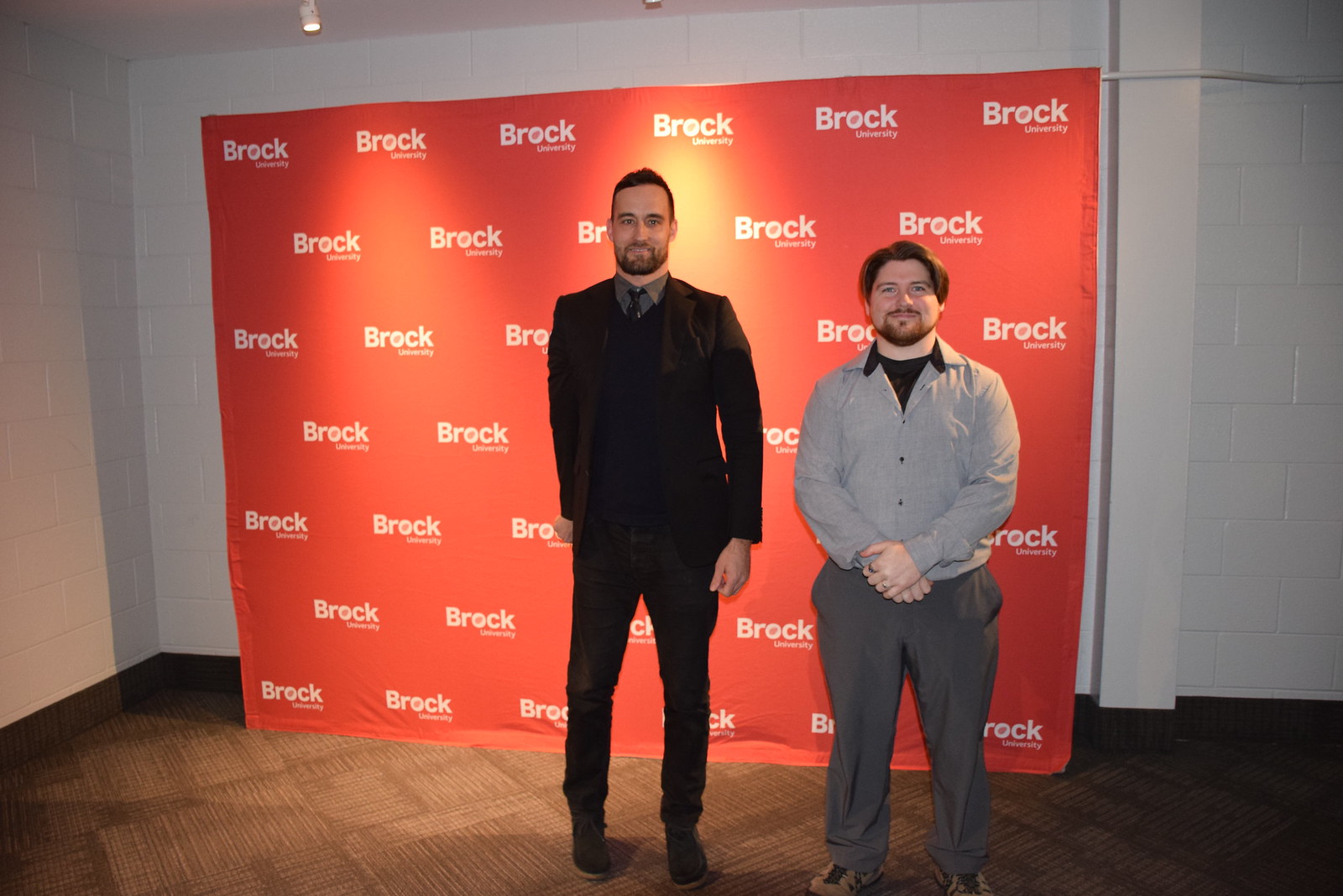In the image, two bearded men are posing in front of a large orange banner with "Brock University" written repeatedly in white letters. The taller man on the left is wearing a dark suit with a black tie and a black sweater underneath, and he stands with his hands awkwardly at his sides. The shorter man on the right is dressed in a gray dress shirt with a black collar, gray slacks, and a black t-shirt underneath. He stands with his hands folded in front of him and is smiling. Both men are Caucasian. They are standing in a room with a plain white wall and brown carpeting. A yellow-glowing, cylinder-shaped ceiling light is visible at the top left of the image.